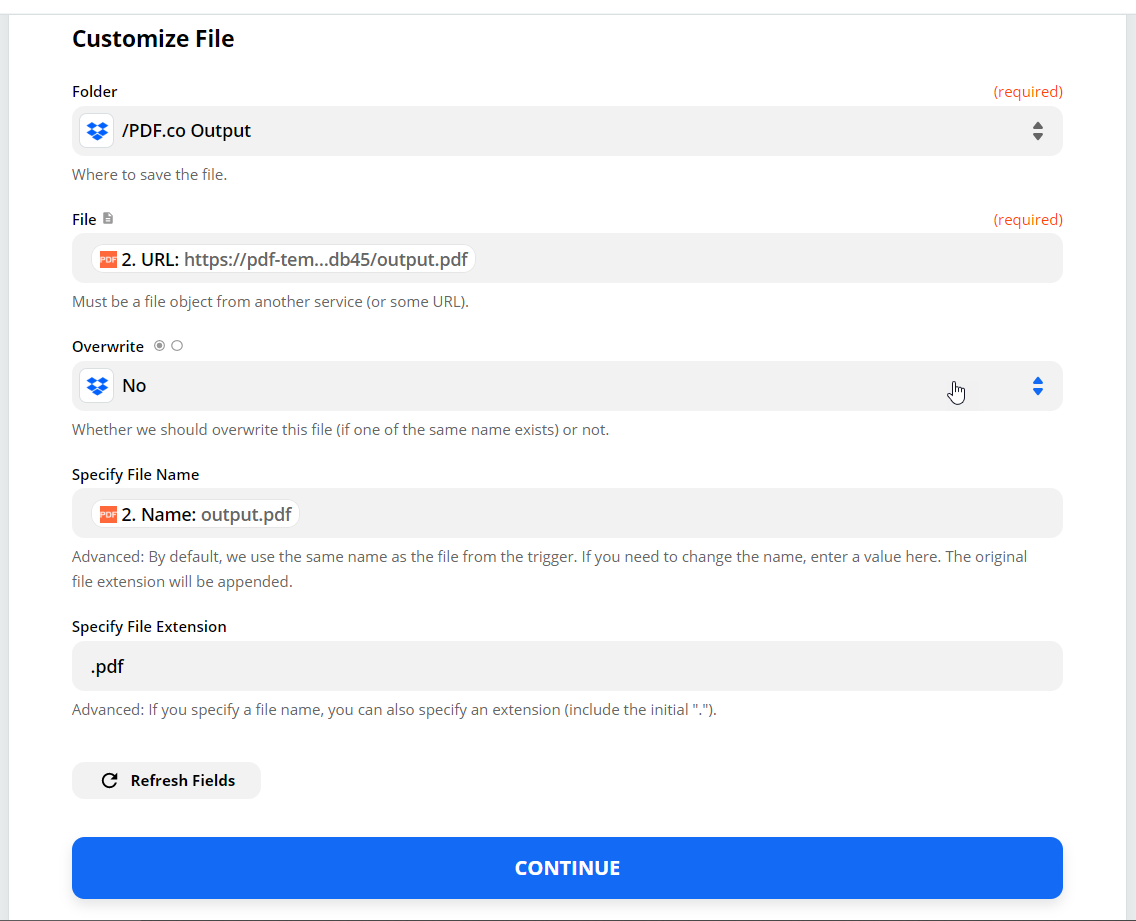A detailed caption describing a website background customization interface:

"This screenshot showcases a semi-programming interface designed for customizing website backgrounds. At the top-left corner, the interface begins with a label 'Customize File' displayed in black font. Directly below this label is a folder icon attached to a gray rectangular bar with a dropdown menu, allowing users to select a specific folder for file customization. The subsequent gray rectangle is a file selection box where users can pick a file and input the desired URL. Below this, there is an option to overwrite or not, enabling users to test their changes in a sandbox environment before committing them to the system. Following this, another gray box provides an area to specify and modify the file name. Adjacent to this is yet another box for determining the file extension. Finally, at the bottom of the interface, there is a prominent blue 'Continue' button that users can click to proceed with the customization process."